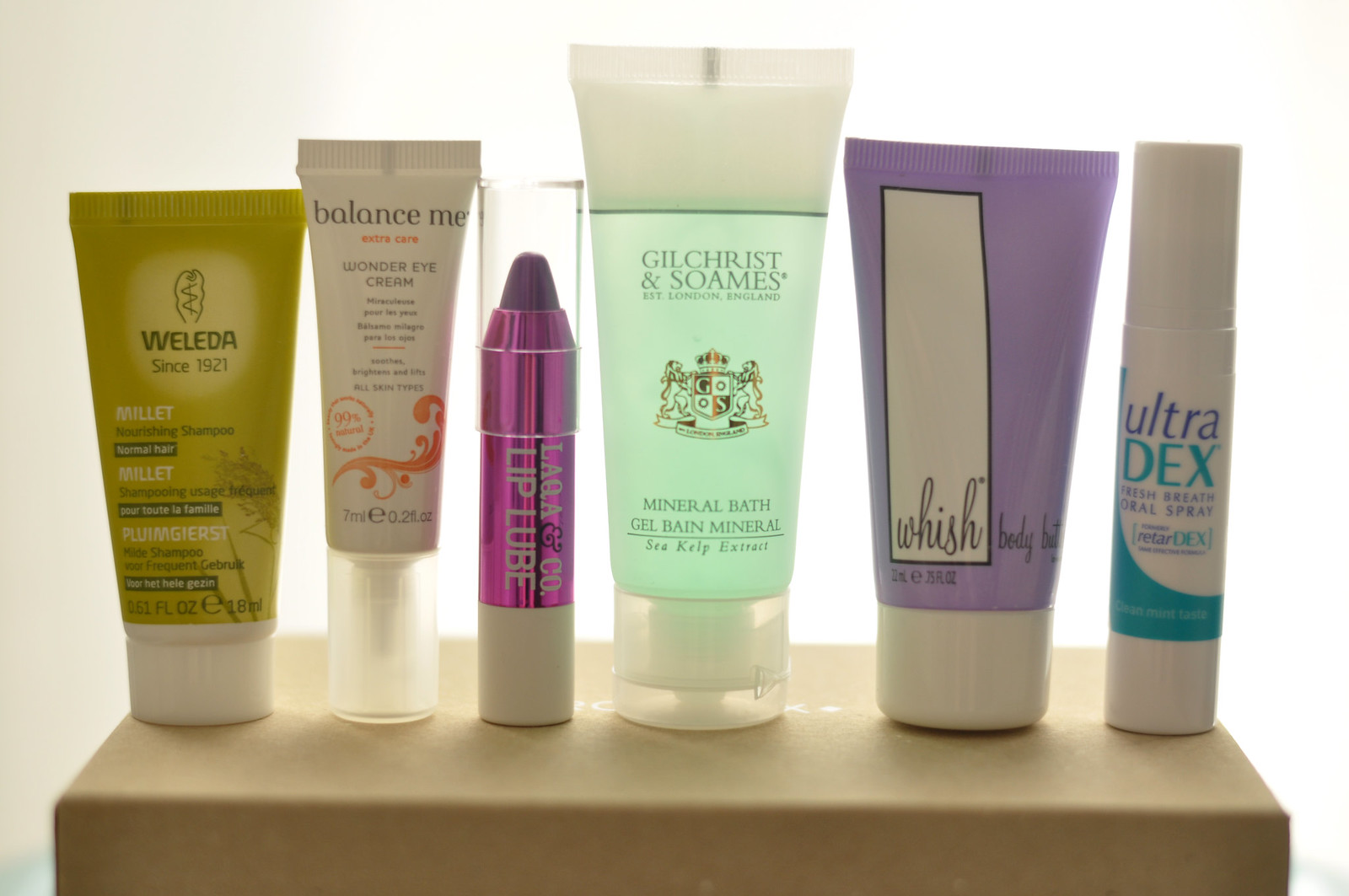A small brown or tan shelf neatly displays an assortment of beauty and personal care products from various brands, reflecting a diverse collection. At the forefront is a bottle labeled "Weleda, since 1921," specifically their "Millet Nourishing Shampoo," designed to pamper hair with its enriching formula. Adjacent to it is a tube marked "Balance Me Wonder Eye Cream," promising to revitalize the under-eye area. Adding a splash of color is the Leo and Company "Lip Lube," a striking purple lip balm to keep lips hydrated. The collection also includes a tube of "Gilchrist and Soames Mineral Bath," offering a luxurious bathing experience. Another tube, albeit with partially obscured text, is labeled "Wish Body," suggesting a skincare product aimed at enhancing one's body care regimen. Lastly, an "Ultradex Fresh Breath Oral Spray" stands ready to ensure minty fresh breath on the go. Each item forms part of a curated selection aimed at head-to-toe care.